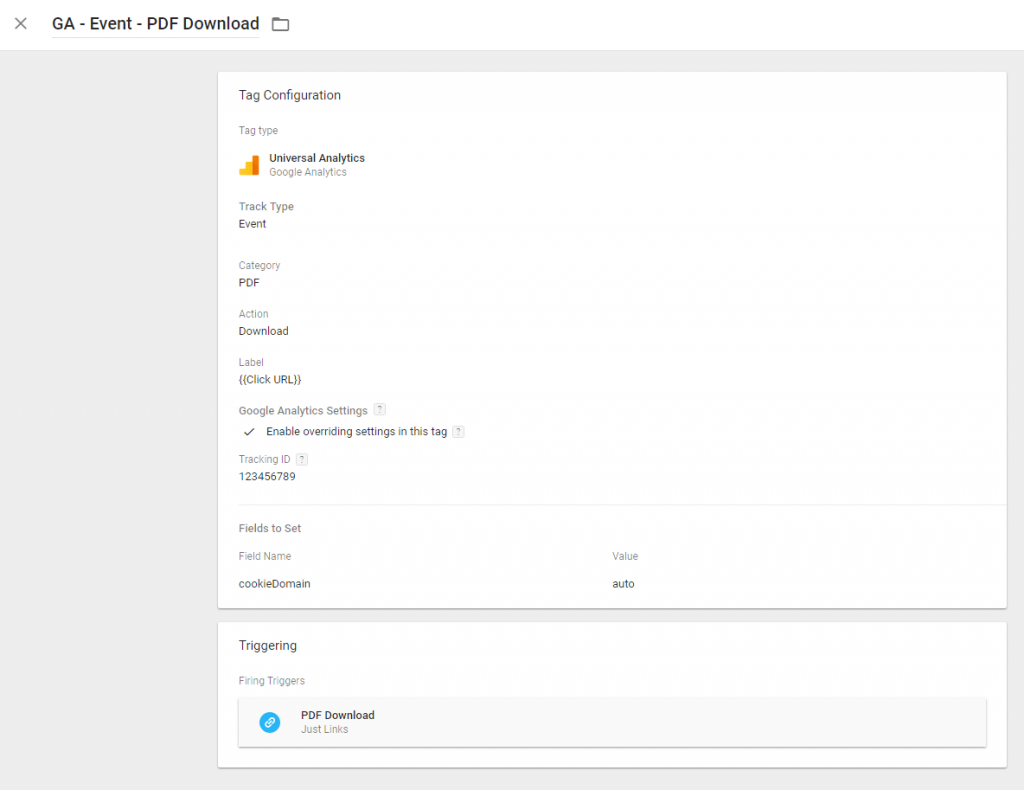The image depicts a computer interface likely related to Google Analytics and tag management. At the top, there is a gray header bar with an 'X' icon in the left corner, followed by three bold labels: "GA", "Event", and "PDF Download." The "PDF Download" label is accompanied by a file icon.

Beneath the header, the interface is divided into two sections. On the left side, there is an empty gray box. On the right side, there is a detailed white box titled "Tag Configuration."

At the top of the white box, it says "Tag Type." Below this, there is a yellow and orange graph indicating data flow, starting small and increasing in size, with the orange section being larger. This section is labeled "Universal Analytics" in black lettering.

Further down, under the "Google Analytics" heading, the following configurations are detailed:
- "Track Type": Followed by an empty line.
- "Event" in bold black lettering: Followed by an empty line.
- "Category": Followed by an empty line, with "PDF" in bold black lettering.
- "Action": Underneath, it says "Download" in bold black lettering.
- "Label": Followed by "Click URL."

Below "Google Analytics Settings," there is a checkbox labeled "Enable overriding settings in this tag," which is checked. Further down, there is a field labeled "Tracking ID" with the value "123456789" in bold black lettering. Lastly, there are fields to set, including "Field Name" and "Cookie Domain," indicating that this configuration could be exported or saved as a PDF file.